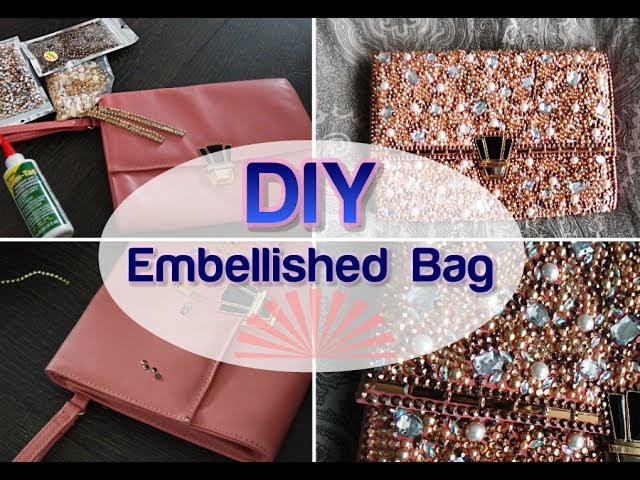The image is an advertisement showcasing a DIY project for embellishing a handbag, divided into a 2x2 grid of photographs with a white, semi-transparent oval in the center that reads "DIY Embellished Bag." In the top left and bottom left photos, there is a square, pink leather clutch with a clasp in the middle, lying on a dark wooden surface. Adjacent to the clutch in the top left image, there are bags of rhinestones and a bottle of glue with a green and yellow label and an orange cap. The bottom left image shows a close-up of the same pink clutch with a few rhinestones and beads being attached. The top right photo depicts the finished product—a pink clutch now fully encrusted with decorative rhinestones and jewels in various colors, including rose gold, red, white, and teal, set against an off-white cloth background. The bottom right photo provides a detailed close-up of the meticulously placed jewels, emphasizing the decorative patterns along the edges of the purse.